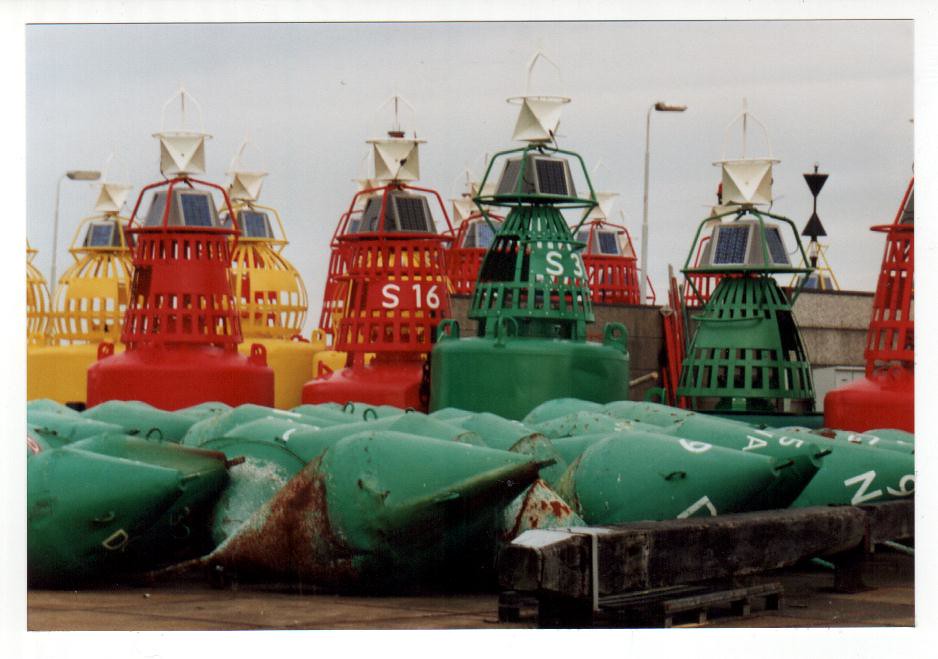The image depicts a collection of variously colored buoys, specifically designed for marine navigation. The scene is shot from the shore and the image is around 20-30% wider than it is tall. In the foreground, there are at least 20 buoys lying laterally on a concrete surface. These buoys are predominantly green and appear to be made of steel, showing signs of rust on their lower sides. Each has a number painted in white, such as "S16" on a red buoy and "S3" on a green one. These lay side by side, in a couple of rows.

Behind the laid-down buoys are other buoys standing upright, painted in red, yellow, and green. These standing buoys are equipped with solar panels and capped with four-sided silver lights, topped off by small radar dishes made up of several triangular segments. A street lamp is visible in the background. The overall condition of the standing buoys is better compared to the rusted ones laying down. The day appears to be overcast, adding a muted tone to the image. The consistent repeated details among the descriptions emphasize the arrangement, colors, and identifying numbers of the buoys as well as their associated equipment.